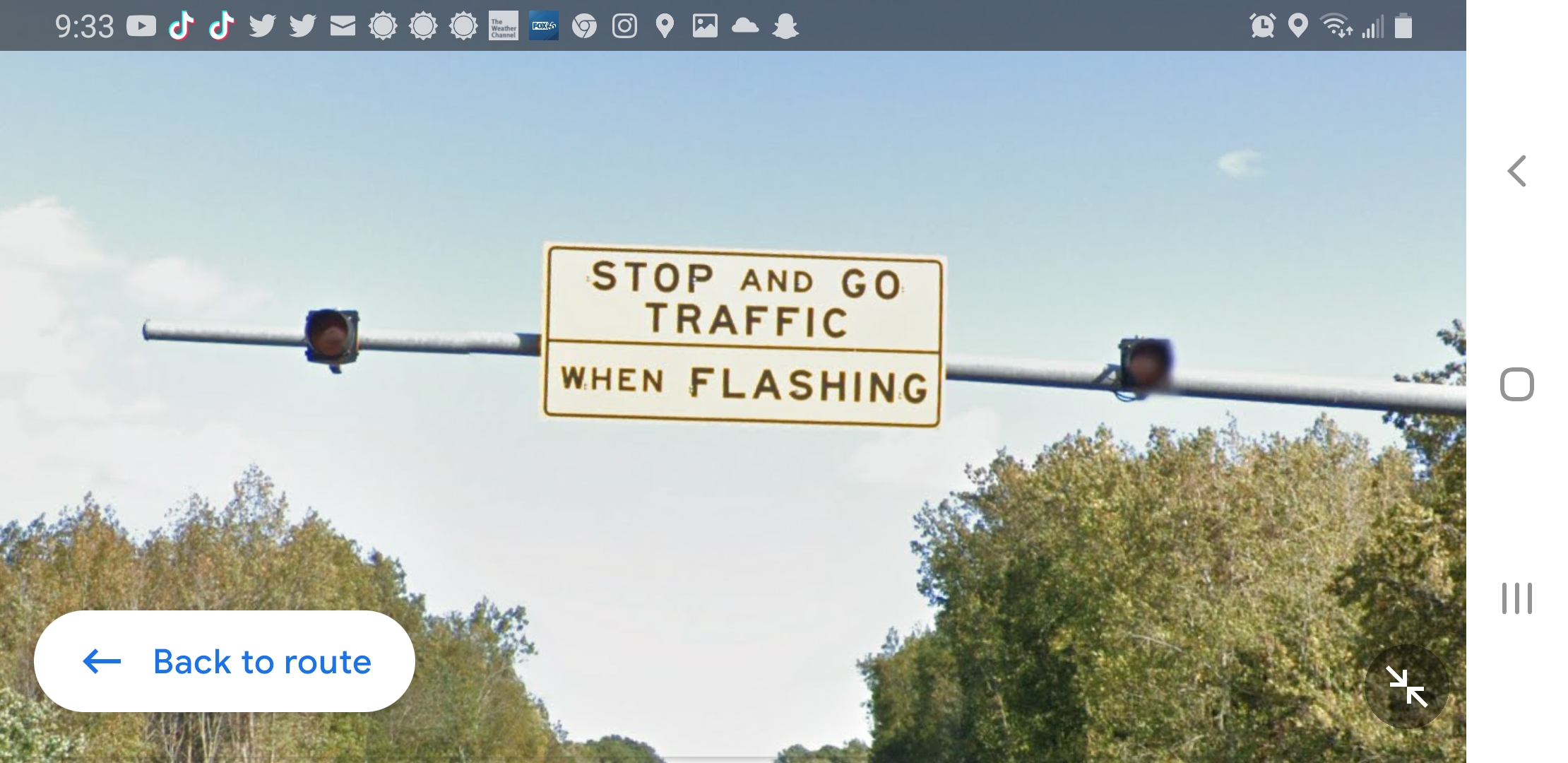This is an image of a traffic sign over a street held on a silver pole and captured in a computer screen image. The sign features two black, square-shaped lights that likely flash red, though they are currently off. Between these lights is a white rectangular sign that reads "Stop and Go Traffic When Flashing" in black lettering. Behind the sign, there are two circular-topped trees with green leaves, set against a clear blue sky speckled with small, indistinct white clouds. On the displayed screen, the top edge shows a dark gray bar listing various notifications, including icons for YouTube, Twitter, TikTok, email, and weather updates, with the time displayed as 9:30. The screen's bottom left corner features an elongated blue oval button that reads “Back to Route” with a left-pointing arrow, suggesting navigation options, and in the bottom right corner, there is a circular icon with two white arrows indicating a zoom function.